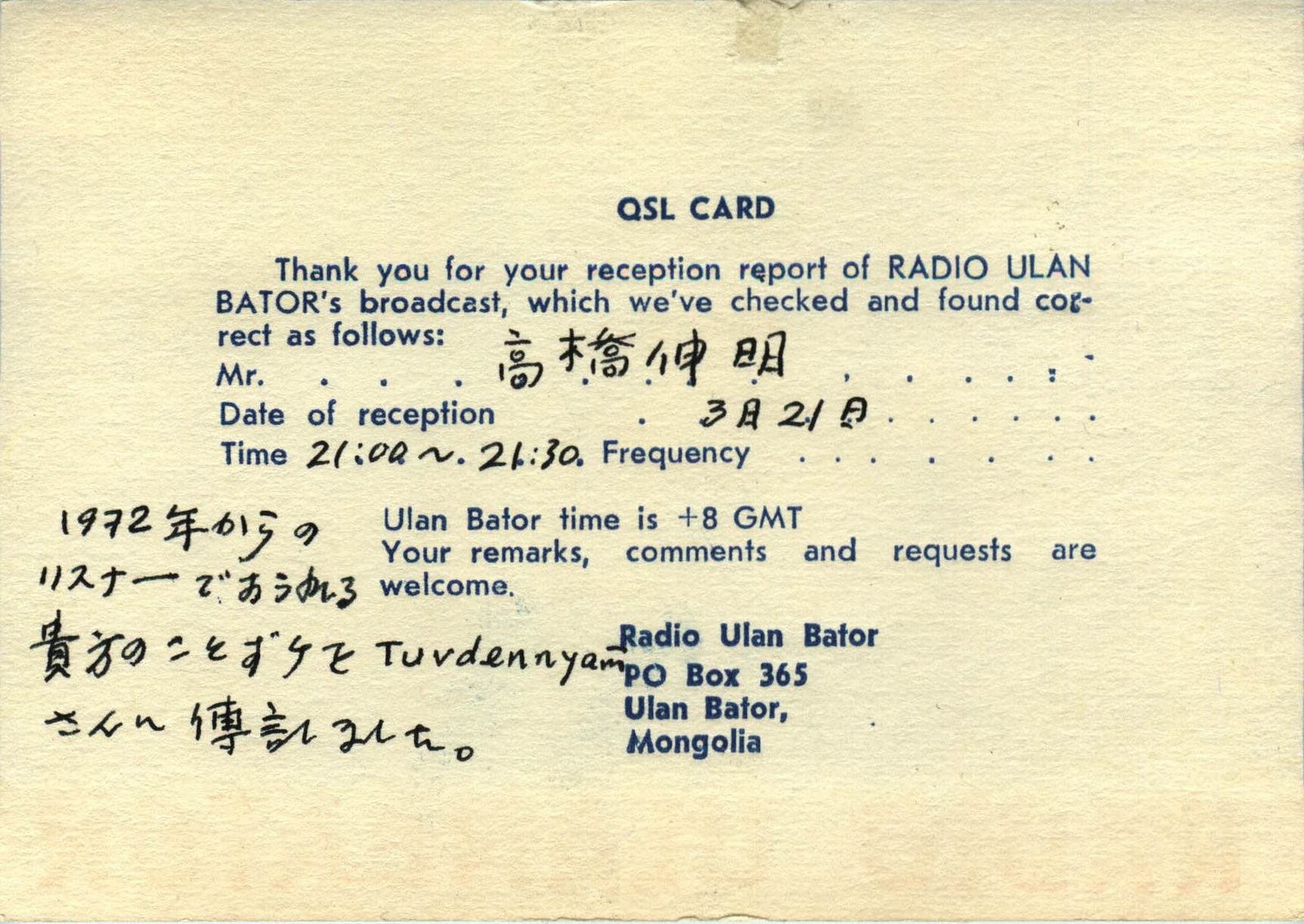This image showcases an aged, cream-colored QSL card with noticeable yellowing, likely indicating its vintage nature. The card features a mix of blue printed and black handwritten text. At the top, in bold blue letters, it prominently displays “QSL CARD.” Below this, it reads, “Thank you for your reception report of Radio Ulan Bator's broadcast, which we've checked and found correct as follows.” The sections for "Mr.," "Date of reception," and "Time" are printed in blue, with handwritten entries in black ink. Next to "Mr.," there is a series of Chinese characters. The "Date of reception" section includes both Chinese characters and a handwritten entry for the time recorded as 2100 to 2130 hours. Additional Chinese characters are dispersed across the card. There's a note indicating that Ulan Bator time is plus 8 GMT, and it welcomes any remarks, comments, and requests from the recipient. At the bottom right, the card provides the station's address: "Radio Ulan Bator, P.O. Box 365, Ulan Bator, Mongolia." On the left side, there are additional rows of Chinese handwritten text, further adding to the card’s rich historical and cultural context.